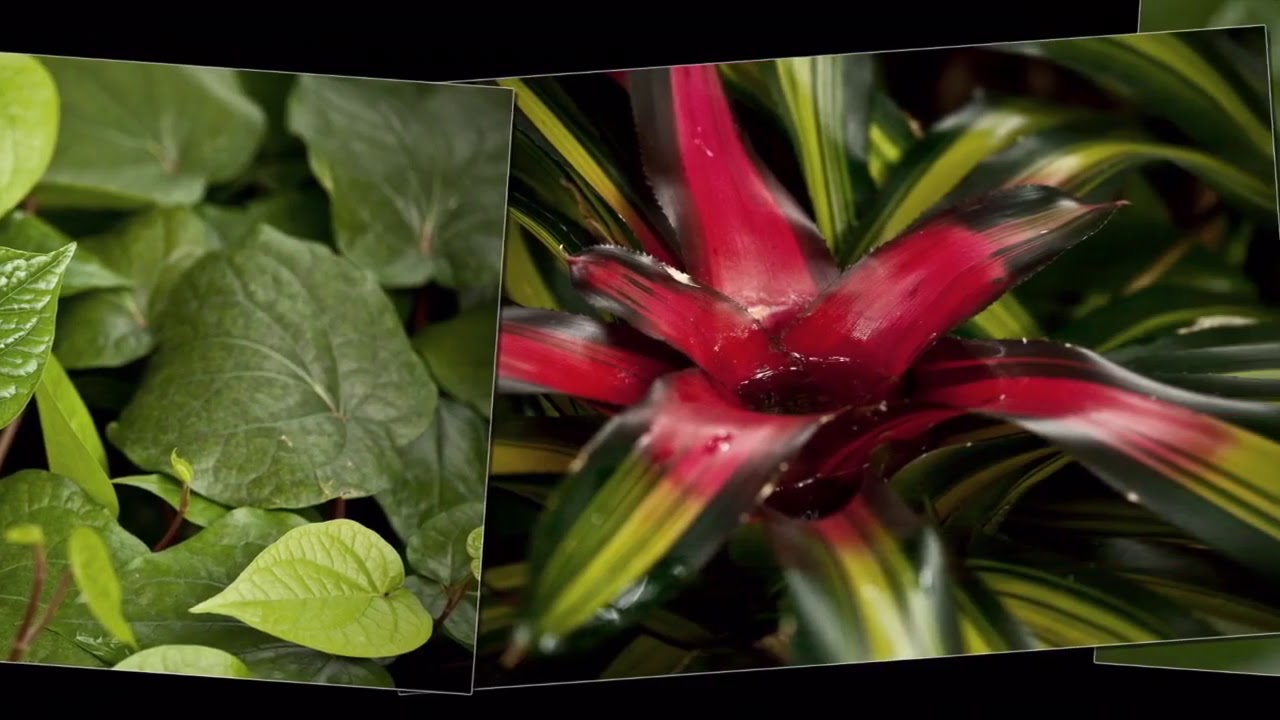The image is a wide rectangular composition showcasing three overlapping images arranged diagonally. The background is a solid black, providing striking contrast. The first image, located on the left side, extends outward with a slight downward curve. It displays a close-up of interspersed dark green and light green leaves, blending together in a compact formation. These leaves vary in size; the larger ones exhibit a deep green hue and an oval shape, while the smaller leaves are lighter green, with a rounded body tapering to a pointed tip.

The second image, placed below the first one and angling upwards toward the top right corner, features a vibrant flower-like plant. This plant boasts thick, pointed leaves with a gradient of colors. The leaves start with a bright red at the center, which then transitions into a dark green at the tips. The central area of the flower is a striking red, accentuating the layered green leaves surrounding it. The plant's intricate structure adds depth and vibrancy to the composition, capturing the viewer's attention.

Together, these overlapping images create a complex visual narrative of lush green foliage and vivid flowering, emphasizing the diversity and beauty of plant life. The entire composition stands upright against the black backdrop, with visible brown stems or roots anchoring the plants to the base of the image.